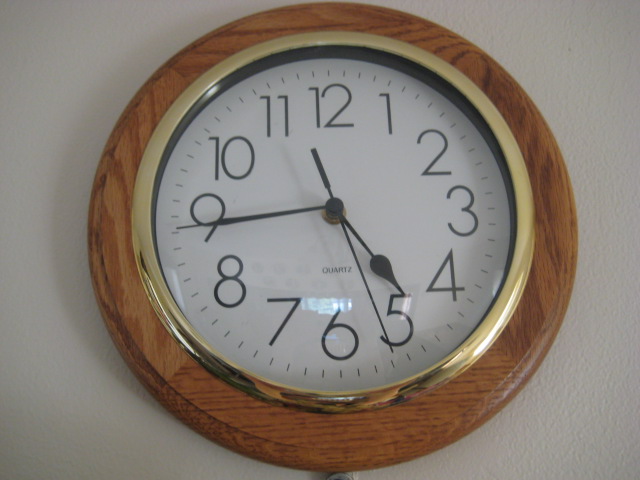This close-up photo features a round wall clock against a white wall that appears slightly dim due to poor lighting. The clock has a medium-toned wood-grain frame encircling a gold metal trim, which in turn surrounds a white clock face. The face of the clock is marked with sixty small tick marks and bold numerical digits from 1 to 12. The time shown is 4:44, with the second hand positioned two notches past the 5. The clock's glass or plastic surface catches a small reflection at the bottom, with another gleam visible on the metal trim to the right.